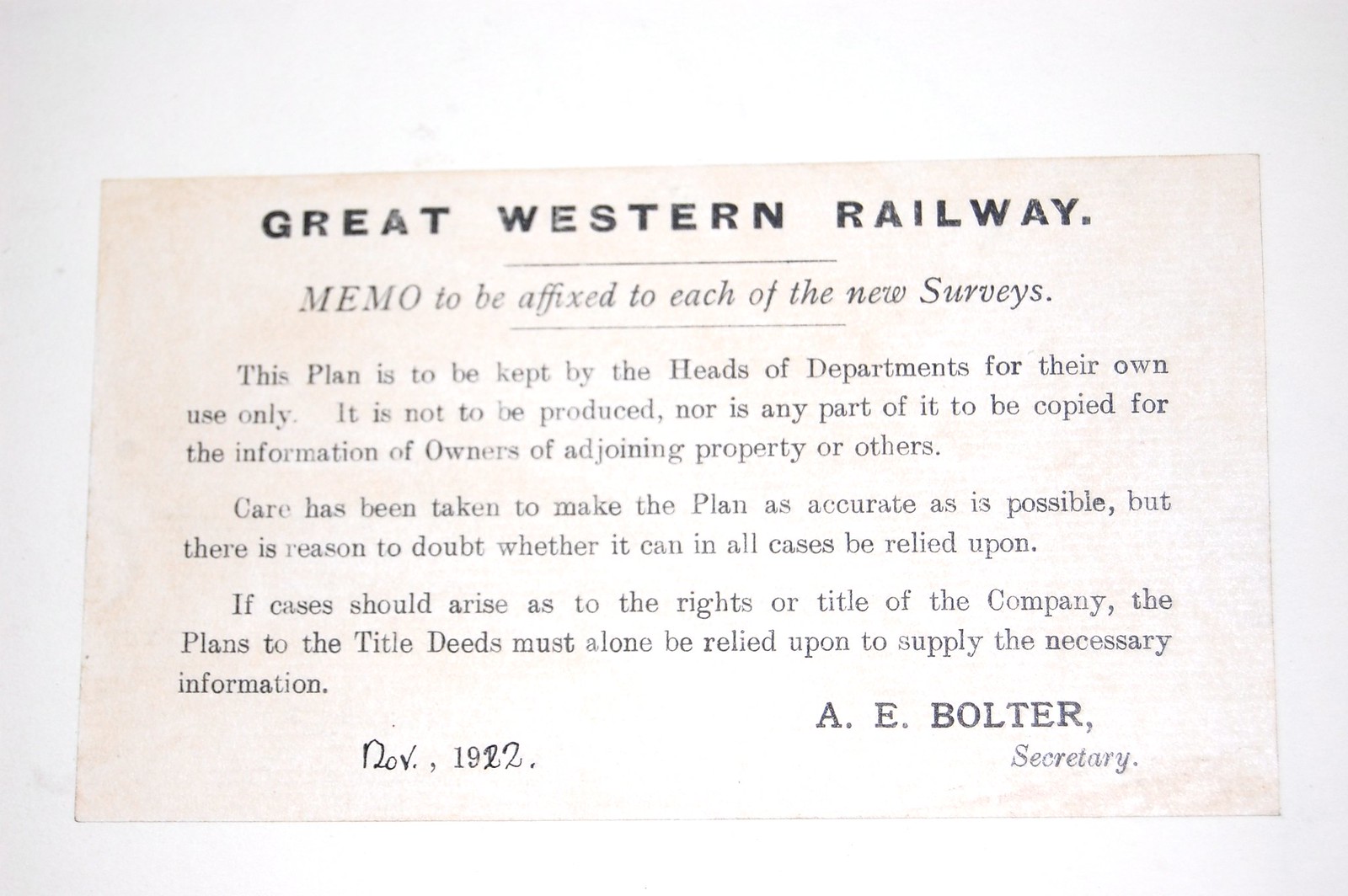This horizontally aligned rectangular image, resembling an index card or piece of paper, features a gray background. At the very top, in bold, all-caps black letters, the title "GREAT WESTERN RAILWAY" is prominently displayed. Directly beneath this, in slightly lighter black text, the memo states, "Memo to be affixed to each of the new surveys." The body of the text is centered on the card and reads, "This plan is to be kept by the heads of departments for their own use only. It is not to be produced nor is any part of it to be copied for the information of owners of adjoining property or others. Care has been taken to make the plan as accurate as is possible, but there is reason to doubt whether it can in all cases be relied upon. If cases should arise as to the rights or title of the company, the plans to the title deeds must alone be relied upon to supply the necessary information." Handwritten at the bottom is "November 1922," and the memo is signed in the lower right-hand corner, "A.E. Bolter, Secretary."